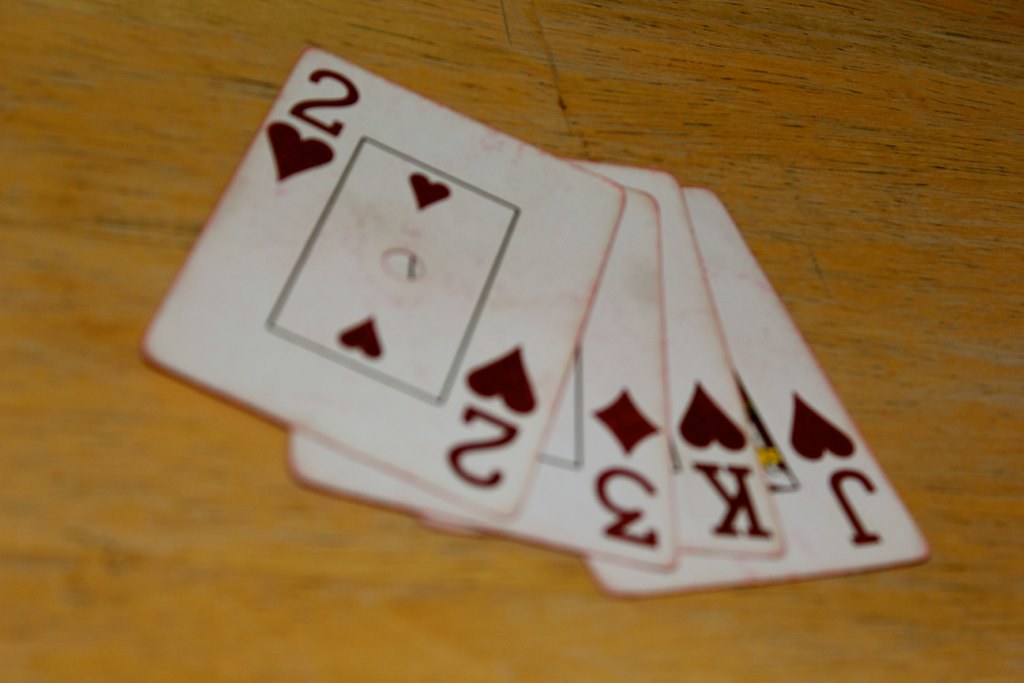A close-up view showcases a hand of playing cards spread on a well-worn wooden table. The table, with its light brown hue interspersed with patches of yellow, exhibits signs of age and frequent use. Four cards are arranged face up, revealing their details. The first card is a Joker adorned with a whimsical hat symbol. Next, a King of Spades stands out with its distinguished black hat symbol. The third card is the Three of Diamonds, identified by its red diamond symbol. Overlapping partially above the other cards, the fourth card is a Two of Clubs, marked with a hat symbol.